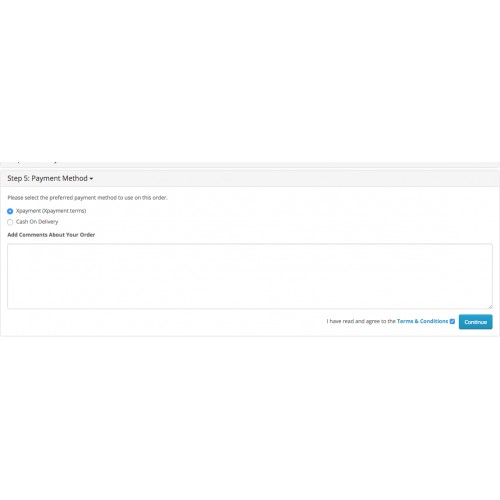This screenshot captures a segment of an online order process focused on selecting a payment method. At the top of the page, "Step 5, Payment Method" is prominently displayed as a heading. Directly underneath, a prompt invites the user to choose their preferred payment method for completing the order. Two payment options are visible: "Payment Current" and "Cash on Delivery," each accompanied by a selection button. 

Beneath the payment options, a text box labeled "Add Comments About Your Order" allows users to input any additional comments or special instructions related to their order. At the bottom right of the page, a checkbox labeled "I Have Read and Agree to the Terms and Conditions" is present, with a hyperlink to the full terms and conditions. Next to this checkbox is a blue "Continue" button, designed for users to proceed to the next step of the ordering process.

The overall layout is minimalist and practical, featuring a white background and black text, with blue accents highlighting interactive elements like the "Continue" button and terms and conditions link. The edges of the screenshot are cut off, indicating that the capture was likely intended to focus solely on the payment method section, possibly for troubleshooting purposes.